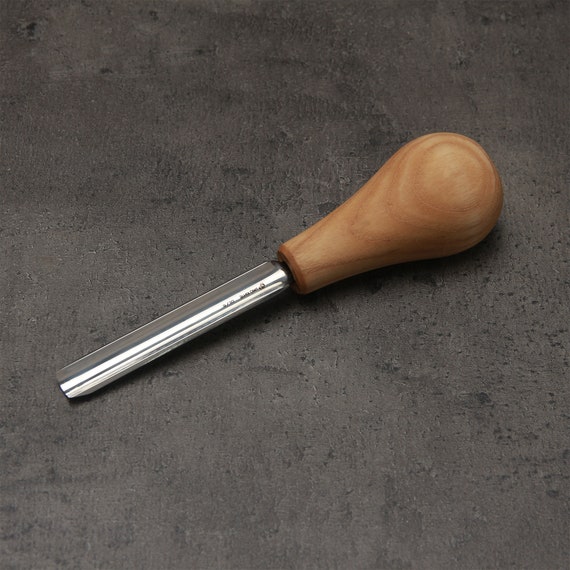The image showcases a wood awl designed for carving, featuring a substantial, bulb-shaped wooden handle made of thick, stained light-colored wood. The handle tapers down towards the base, where it connects to a long, flat metal blade that measures approximately 5 inches in length. The blade is sharp along the edges and appears to be slightly hollowed out in the center, indicative of a tool meant for creating holes or grooves in wood when struck with a wood mallet. The top surface of the metal blade, which reflects light, adds a subtle gleam to the image. Near the base of the metal part, there is a small inscription in black text, though its content is not discernable. The tool is positioned on a gray, pockmarked concrete floor, contributing to the simple, industrial composition of the photograph.